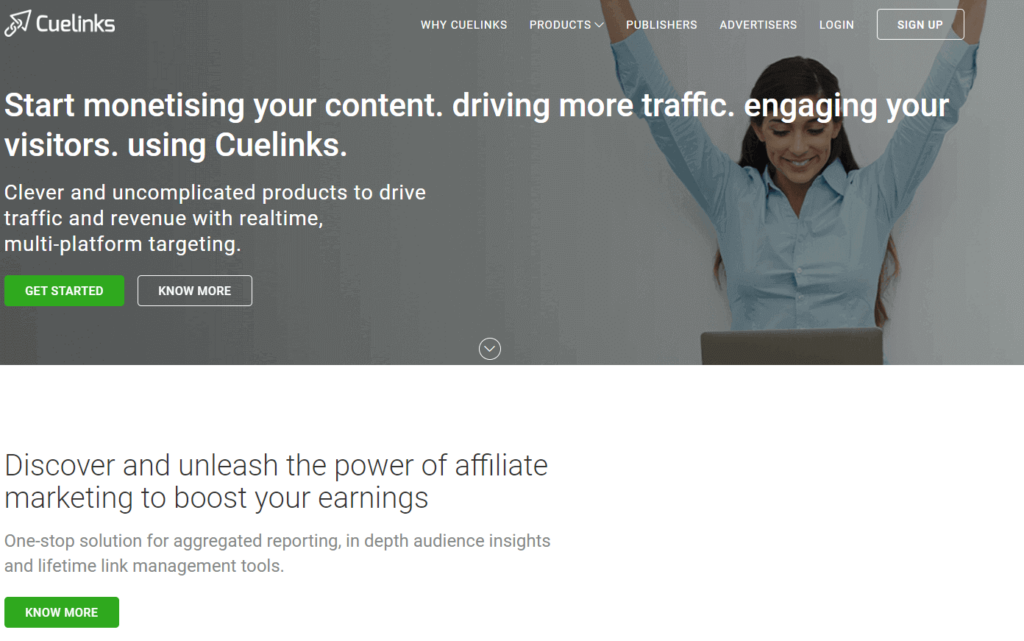In the image, there's a detailed webpage layout displaying various features and functionalities:

1. **Top Menu Bar:**
   - **Q-links:** Represented by an icon featuring a triangle and a link with two circles.
   - **Y-Q-links:** Followed by menu options for **Products**, **Publishers**, **Advertisers**, **Login**, and **Sign-up** which is enclosed in a rectangle.

2. **Main Visual:**
   - A cheerful woman wearing a blue-collared shirt is pictured. She has long hair and has both her hands raised above her head in a gesture of excitement. She is looking at her laptop with a broad smile, showing her teeth.

3. **Promotional Text:**
   - The text overlay says, “Start monetizing your content, driving more traffic, engaging your visitors using Q-links. Clever and uncomplicated products to drive traffic and revenue with real-time, multi-platform targeting.”

4. **Call-to-Action Buttons:**
   - A green rectangle at the bottom center with white text that says, “Get Started.”
   - Below, a gray rectangle with white text that says, “No More.”

5. **Additional Information:**
   - Another descriptive section reads, “Discover and Unleash the Power of Affiliate Marketing to Boost Your Earnings. One-Stop Solution for Aggregated Reporting, In-depth Audience Insights, and Lifetime Link Management Tools."

6. **Additional Call-to-Action (Repeated):**
   - Another green rectangle with white text that says again, “No More.”

The overall layout is designed to provide a comprehensive understanding of the services offered, with visually engaging elements and clear actionable steps for the user.